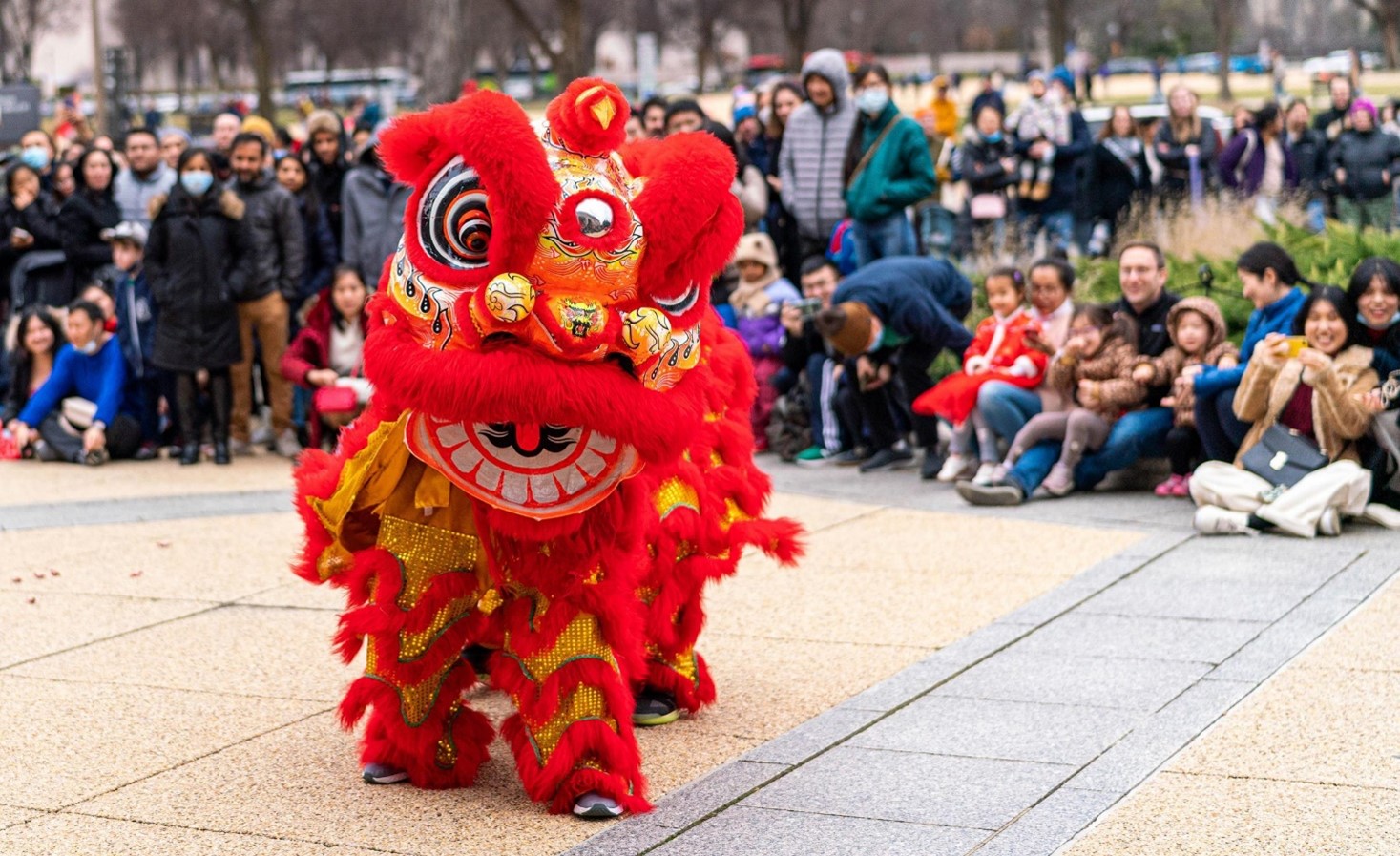The image captures a vibrant outdoor Asian-themed celebration centered around a captivating dragon dance. The scene is set on a tan cement courtyard segmented by a gray strip that runs diagonally from the middle bottom to the right. Dominating the left side of the image is an elaborate dragon costume adorned in rich reds and golds. The dragon's large head features striking spiral eyes with blue, white, and yellow concentric circles and a distinctive red mustache over its open mouth. The costume's legs are decorated with red curvy shapes and gold accents, and you can glimpse the performers' sneakers beneath it.

In the background, numerous onlookers—many clad in jackets suggesting a winter setting—are gathered to watch the performance. The audience appears to include many families, hinting at the event's communal and festive nature. Behind them, a line of trees further enhances the park-like atmosphere. The overall scene depicts a cultural celebration brimming with color, movement, and shared enjoyment.